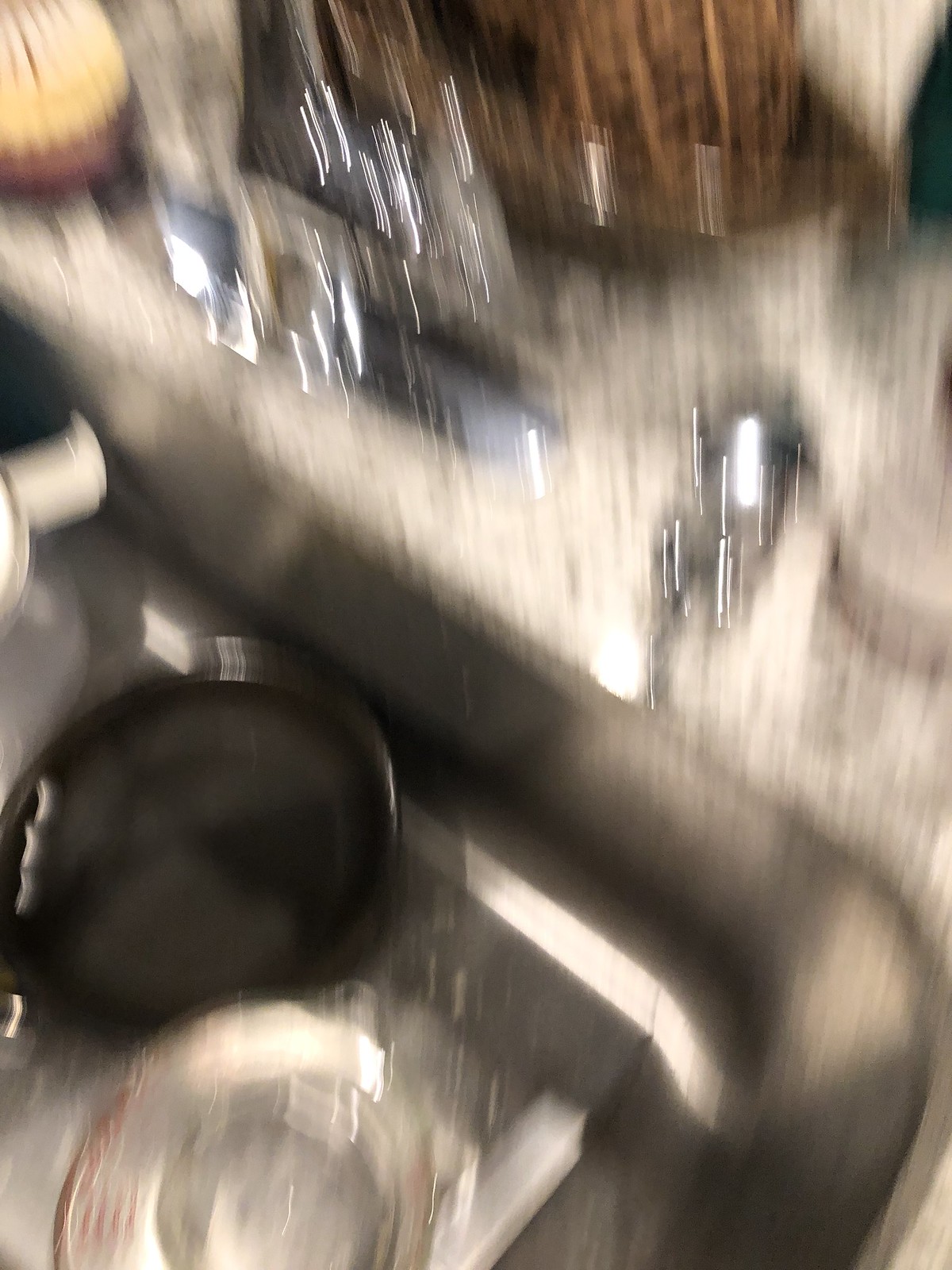On a kitchen counter made of sleek granite sits an undermount sink, which contains a few items. Among them is a small frying pan and a glass measuring cup. Clustered around the sink are several pieces of silverware. A glass bottle of red hot sauce and various other condiments are placed nearby. In the background, a brown wicker basket can be seen, adding a rustic touch to the scene.